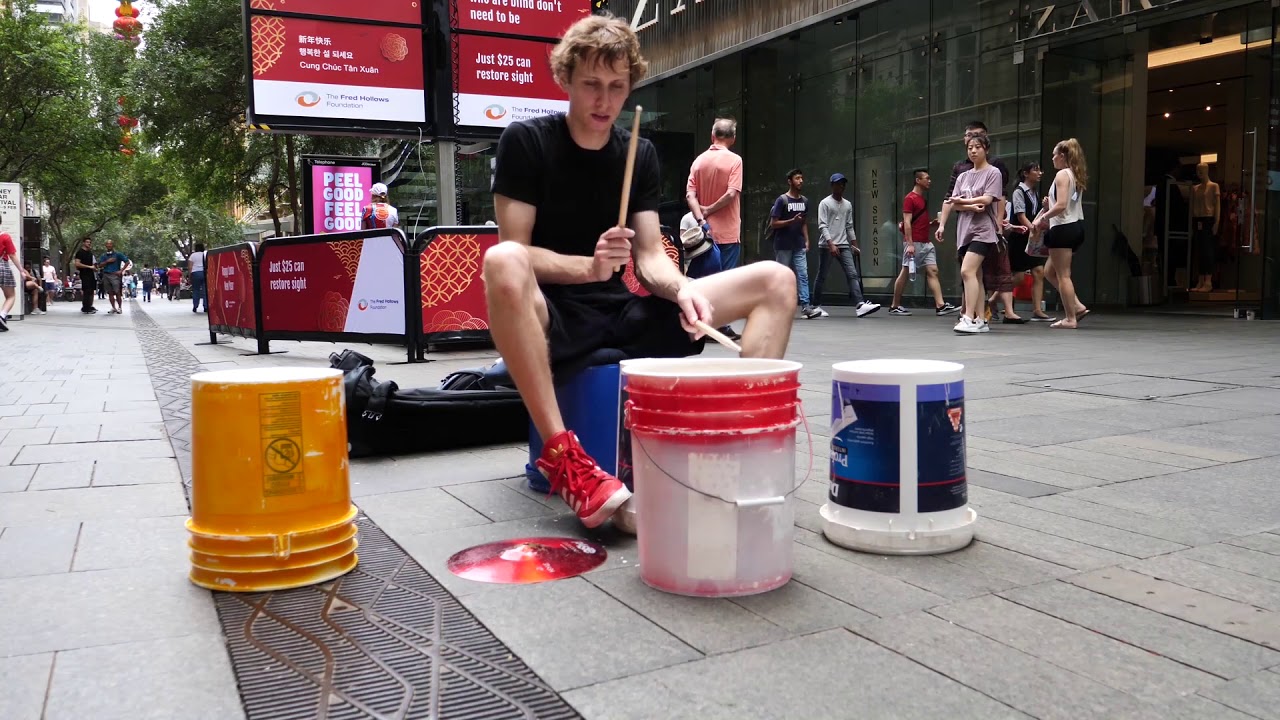A young street performer wearing a black short-sleeve shirt, black shorts, and bright red gym shoes is sitting on a blue bucket at a city street, possibly near a bus stop or metro station. He is playing drums using three brightly colored buckets: one yellow, one white with a red painted rim, and another white bucket with a blue label. He is positioned in front of a white bucket with a red rim. The gray pavement around him suggests a bustling shopping district with people walking by, some of whom appear indifferent while one person in particular looks at him. The wide street in the scene features a grid-like pattern down the middle and a backdrop of trees and overcast sky. Behind the performer, there are signs on a fence with ads, including messages like "Just $25 can restore sight" and "Feel good, feel good." The area gives a lively urban vibe, with a hint that he might be outside a department store or a restaurant.